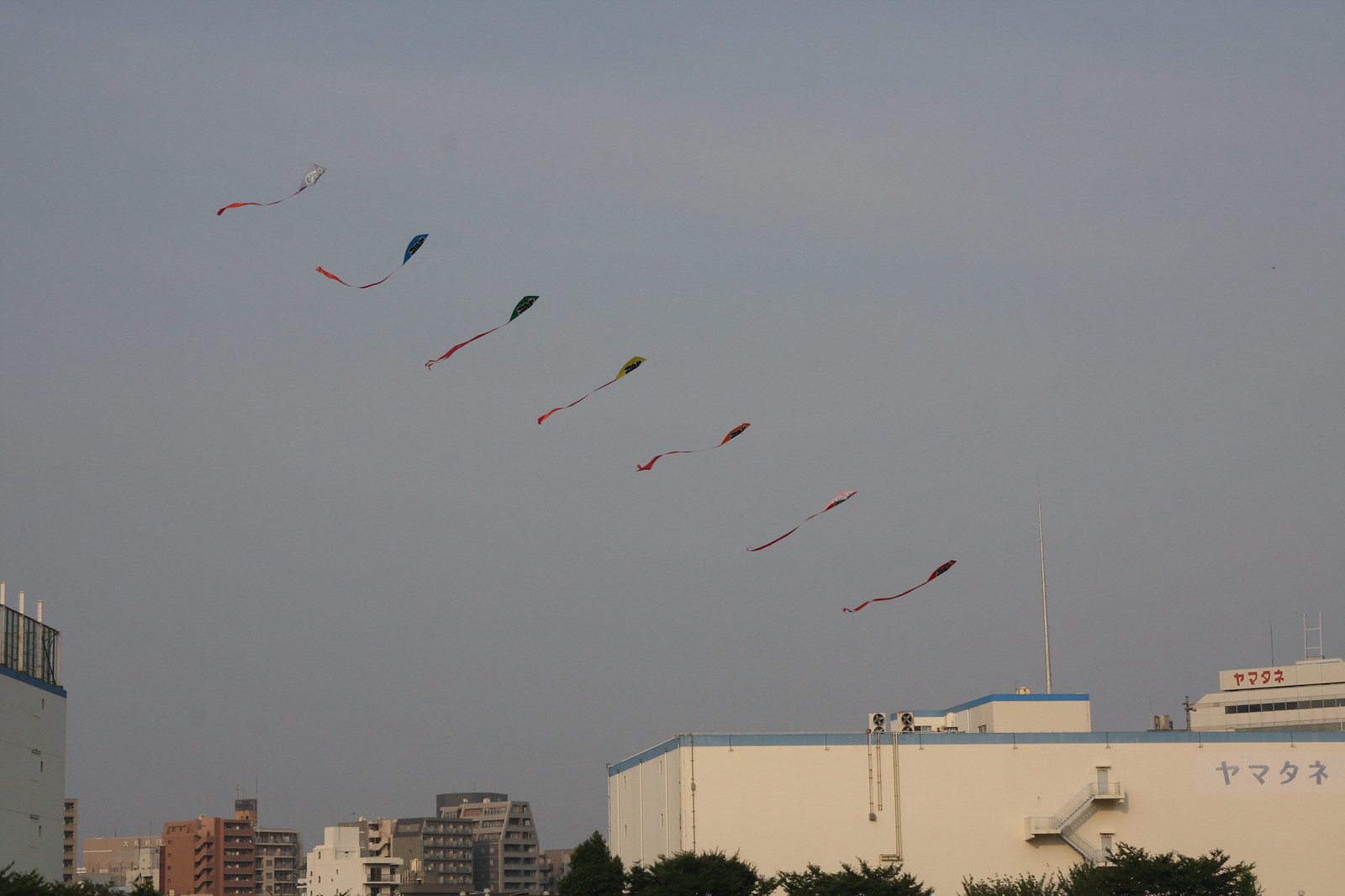The photograph captures a late evening scene outdoors, under a dark and cloudy sky. Dominating the upper expanse of the image are seven kites flying diagonally from the upper left to the lower right, each sporting a long red tail that flutters in the wind. The kites are lined up equidistantly, in a neat and staggered formation, with the highest kite in the upper left corner and the lowest in the bottom right. They vary in color, including blue, green, yellow, orange, gray, and shades of red.

In the foreground, on the lower right, stands a large white building adorned with hiragana, indicating it is likely situated in an Asian country. On the lower left, a series of apartment buildings with numerous small windows and balconies can be seen, contributing to the urban landscape at the bottom edge of the photograph. The sky, despite being overcast, serves as a stark, featureless backdrop for the vibrant kites, creating a compelling contrast.